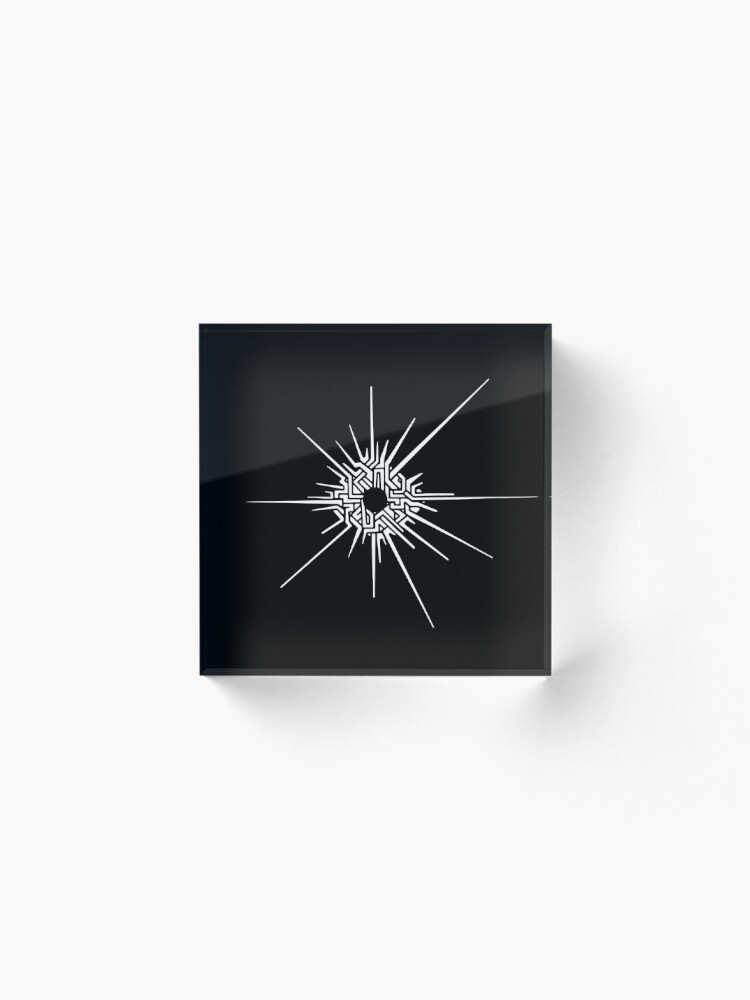The image depicts a framed piece of abstract digital art centered against a pristine white wall. The artwork itself is defined by a glossy black square with a subtle gradient, transitioning from gray at the top to a deeper black at the bottom, creating a striking diagonal contrast. At the heart of the black square is a compelling white starburst or sunbeam pattern radiating outward from a central solid black circle, resembling a shattered glass effect or a maze-like web of tangled lines. The pattern is composed of numerous jagged, spiky lines of varying lengths, weaving an intricate design that evokes a sense of dynamic movement and intricate complexity. The entire aesthetic of the piece combines modern abstract elements with a visually arresting interplay of black and white tones, making it a standout in any art collection or exhibit.